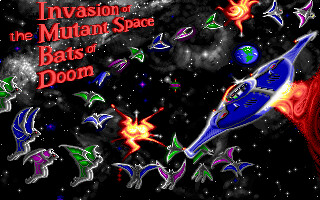This image is a screenshot from an early-style video game titled "Invasion of the Mutant Space Bats of Doom." The screen emulates the aesthetic of vintage handheld or early laptop games, characterized by its very low resolution and pixelated graphics. Dominating the scene are vibrant, simplistic bats rendered in various colors, all possessing rudimentary, jagged edges. On the right side of the screen, a blue spaceship is visible, with its trajectory marked by swirling trails of orange, yellow, and white light, giving a sense of dynamic movement. The backdrop is a dark cosmos speckled with points of light that represent stars, galaxies, and solar systems, adding to the space-themed ambiance. In the upper right corner, a portrayal of Earth is discernible. The game's title, "Invasion of the Mutant Space Bats of Doom," is prominently displayed in a reddish-orange hue in the upper left corner, completing the retro feel of this captivating screenshot.